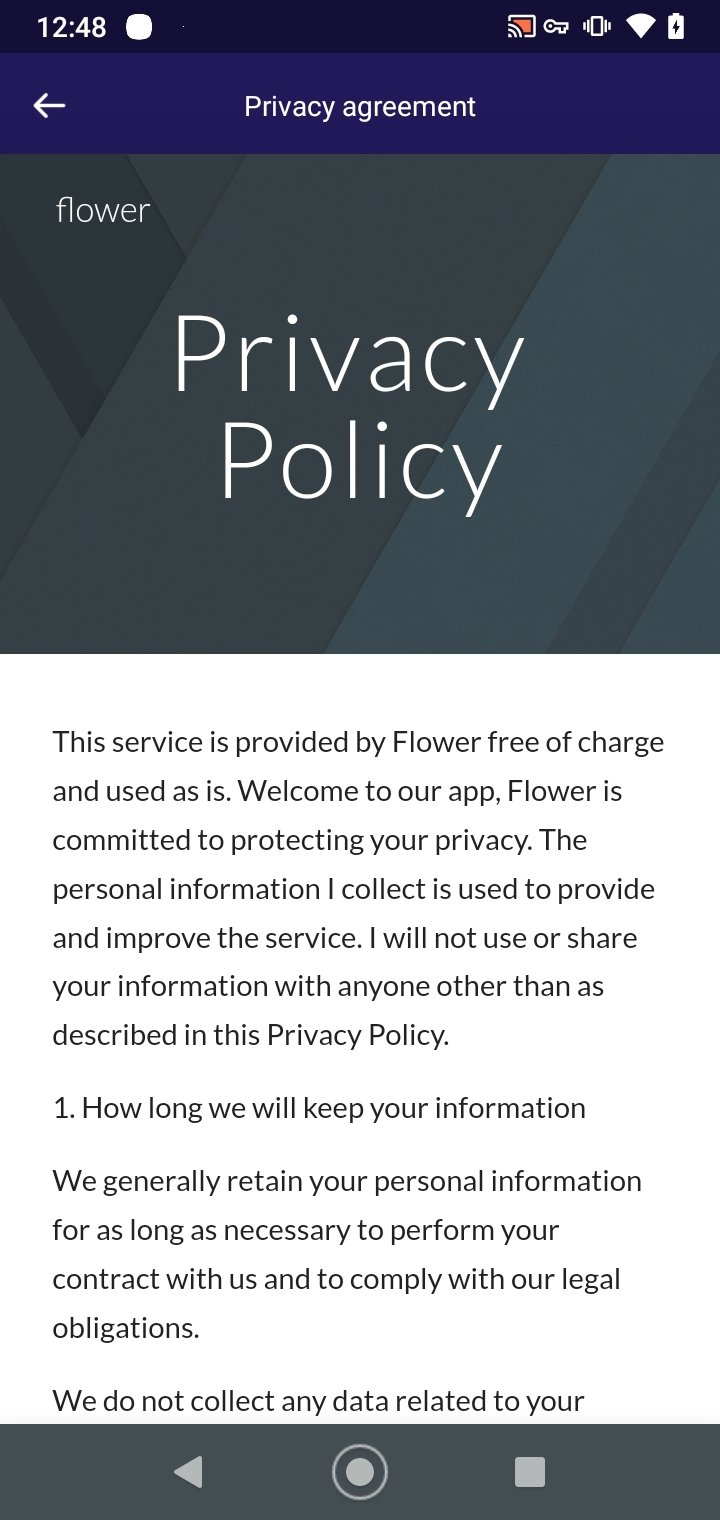**Detailed Caption for the Image**

This image is a mobile screenshot capturing the privacy policy of an application or website, possibly named "Flower." The screenshot was taken at 14:48, as indicated by the time stamp on the top left of the screen. On the top right of the status bar, several icons are visible, including those for battery life and Wi-Fi signal strength, along with three additional, unrecognized icons.

The main interface has a header bar with a purple background, displaying the text "Privacy Agreement" prominently. There is a white arrow on the left side of the header, which appears to be a back navigation button. The text "Flower" is shown below it in a smaller font, followed by a more prominent "Privacy Policy" in larger text.

The body of the privacy policy is set against a white background with black text. It starts with:
"The service is provided by Flower, free of charge, and used as is. Welcome to our app. Flower is committed to protecting your privacy. The personal information I collect is used to provide and improve the service. I will not use or share your information with anyone other than as described in this policy."

It then outlines the retention period for personal information:
"Privacy Policy 1. How long we keep your information. We generally retain your personal information for as long as necessary to perform your contract with us and to comply with our legal obligations."

The text is cutoff towards the end:
"We do not collect any data related to your..."

At the bottom of the screen, the typical mobile navigation bar is visible, featuring the back button, home button, and menu button. The overall design reflects a standard mobile privacy policy page with navigational elements and introductory legal text.